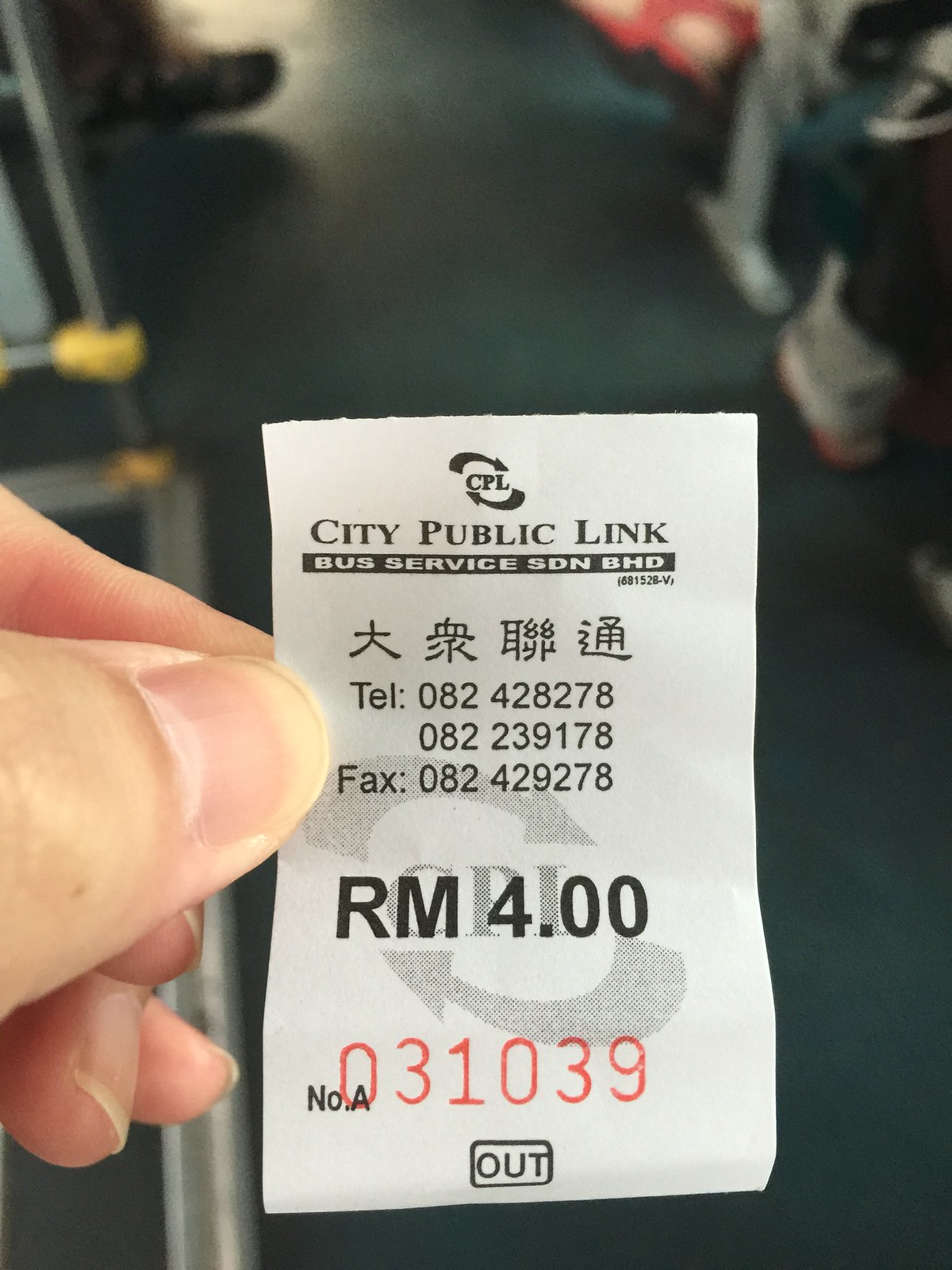This close-up, photorealistic image captures a hand from the left side delicately pinching a small bus ticket between the thumb and pointer finger. The white ticket features a semi-transparent gray logo of two arrows circling the letters CPI in the center, with a smaller black version of the same logo at the top. Just below the black logo, "CITY PUBLIC LINK" is printed in bold, black capital letters, followed by "BUS SERVICE SDN BHD" in white text over a black banner. The ticket further includes foreign characters beneath this banner, followed by a telephone number and a fax number. Below these, the fare is printed as "RM 4.00" in large black font. Additionally, a red-stamped sequence "031039" and the word "OUT" encased in a black box are visible at the bottom. The blurred background reveals green flooring and the indistinct images of shoes, suggesting the setting is inside a bus or some other form of public transportation.